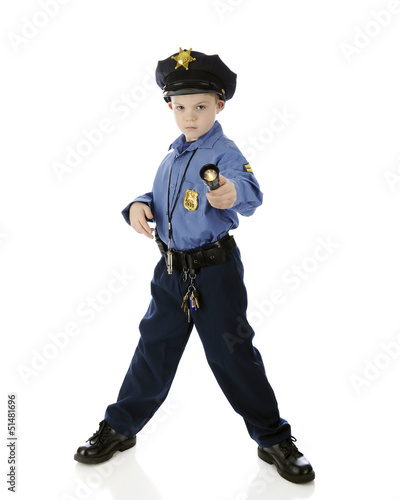A young boy stands in a white, possibly studio setting, dressed in a detailed police costume. He stares intently at the camera, highlighting his serious expression. His attire includes a black police hat with a gold sheriff’s star at the top center, a light blue shirt featuring a gold badge on the left breast and an emblem on his left shoulder, and dark navy blue pants. Around his neck hangs a whistle, while a black belt with keys drapes around his waist. In his left hand, he firmly grasps a black flashlight pointing towards the camera, and his right hand rests at his side. Completing his outfit are shiny black shoes, whose reflection is visible on the gleaming white floor. The image is watermarked with "Adobe Stock" across it and includes the stock number 514-816-96 in the lower left corner. The boy's brown hair, dark eyes, and the meticulous placement of his costume elements suggest a staged photo shoot, possibly for a Halloween or themed event.